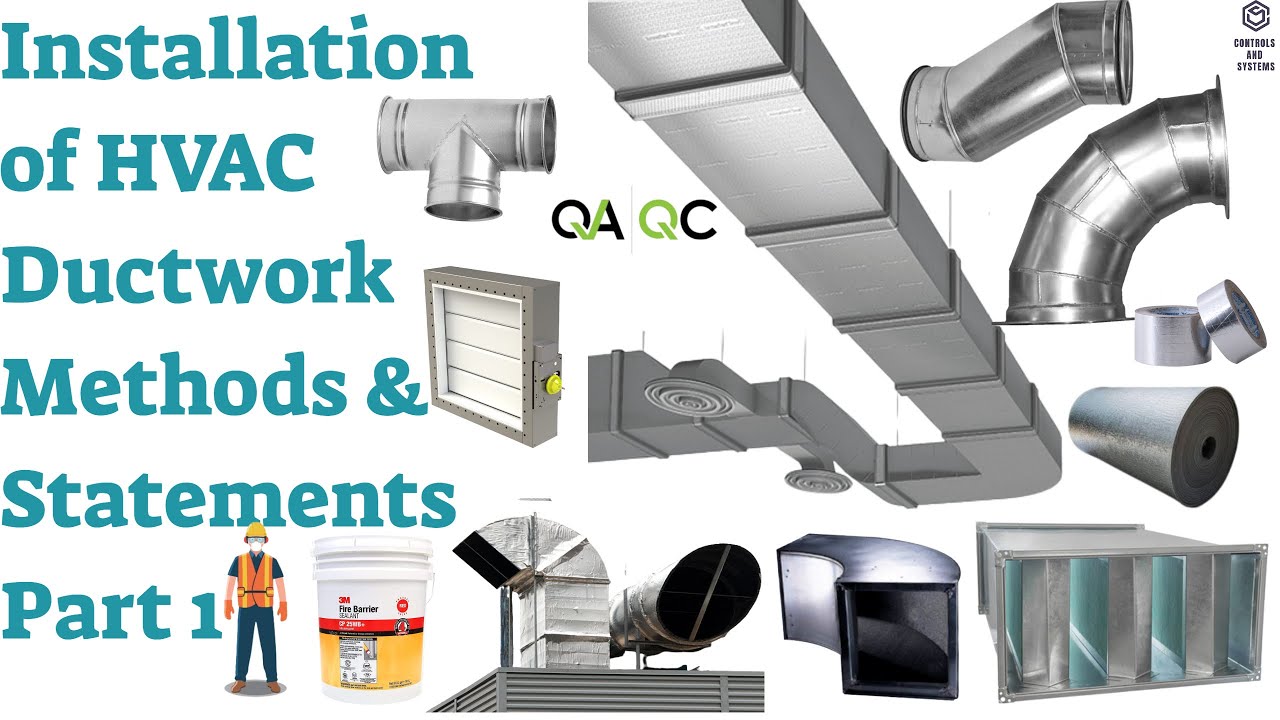The image is a color diagram titled "Installation of HVAC Duct Work Methods and Statements, Part 1," written in blue letters along the left side. Adjacent to the title, there is an illustration of a worker dressed in gray, wearing a yellow and orange vest, orange gloves, a yellow hard hat, orange headphones, and a white mask. To the right of the worker's image is a color photo of a white barrel with red and yellow labeling, indicating it contains 3M Barrier Sealant. The right side of the image displays various types of metal ductwork, including straight and curved sections as well as a vented piece. Interspersed among these images, there are black and green letters spelling out "QA, QC." In the upper right corner, in black lettering, the words "Controls and Systems" are displayed, with a square symbol above it.